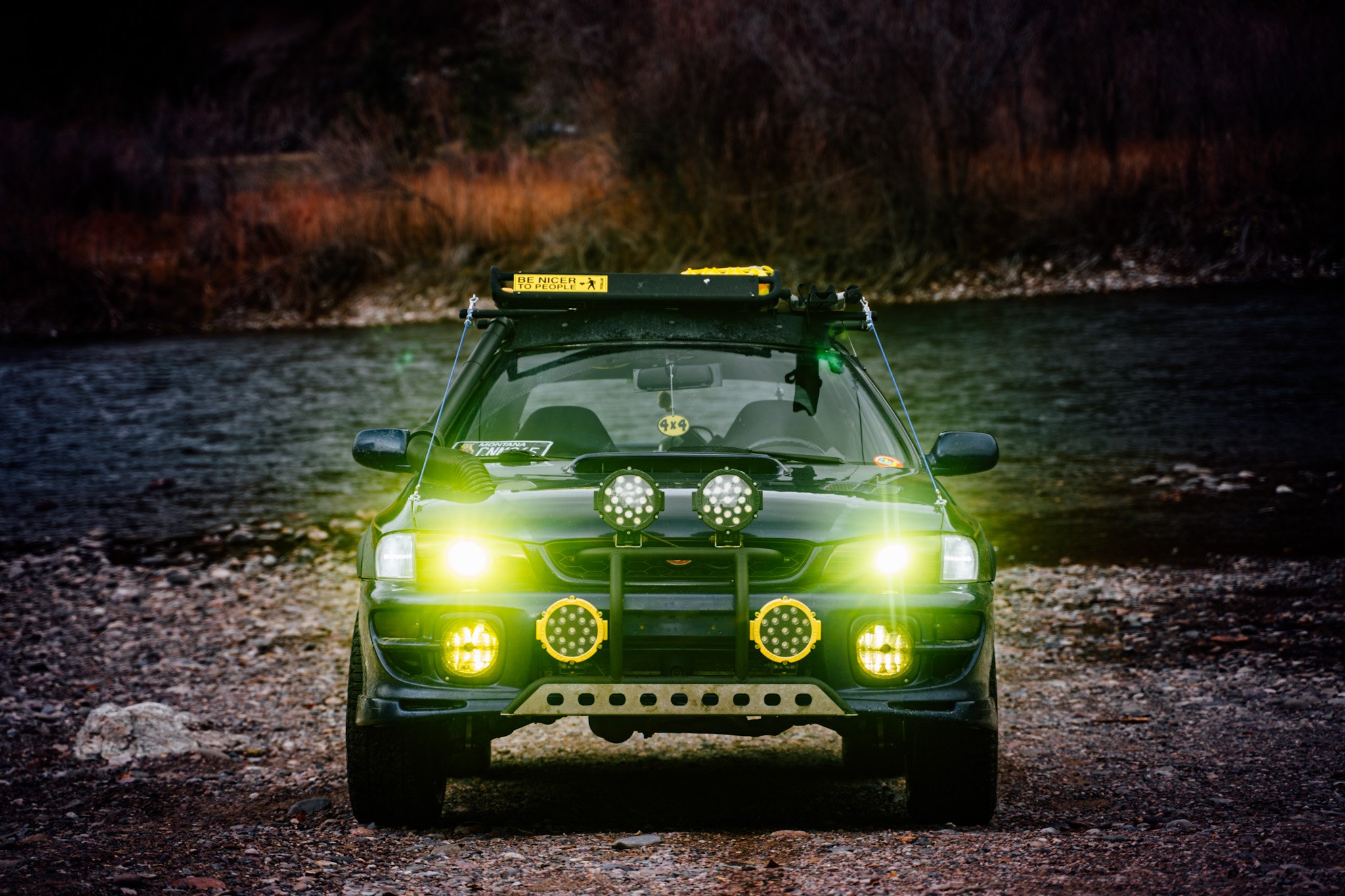In this close-up landscape photograph, we see a black car with a sporty appearance, facing the viewer and positioned on a rough, rocky terrain. The car is equipped with a rack on the roof, designed for carrying objects, and features black seats and tires. Prominently displayed on the vehicle are multiple sets of headlights: the top and bottom sets are yellow and circular, casting a bright light forward, possibly to aid in navigating difficult, low-visibility terrains. Additionally, there are supplemental lights attached to the grill, emphasizing the car's readiness for outdoor adventures or nighttime driving.

The car's bumper is silver-brown and flat, with multiple holes drilled into it, indicating a rugged build. The scene around the car is filled with small, scattered rocks in hues of gray, orange, and reddish-brown. Behind the vehicle flows a large, raging river, with banks lined by rocks and scattered patches of grassland. The grass is a mix of orange and red shades, hinting at an autumn setting. In the distance, blurred and faded trees and another barely visible vehicle complete the background, adding depth to the image. Although the car is in full light suggesting daytime, there are darker edges around the scene, possibly an intentional vignette effect to focus attention on the car.